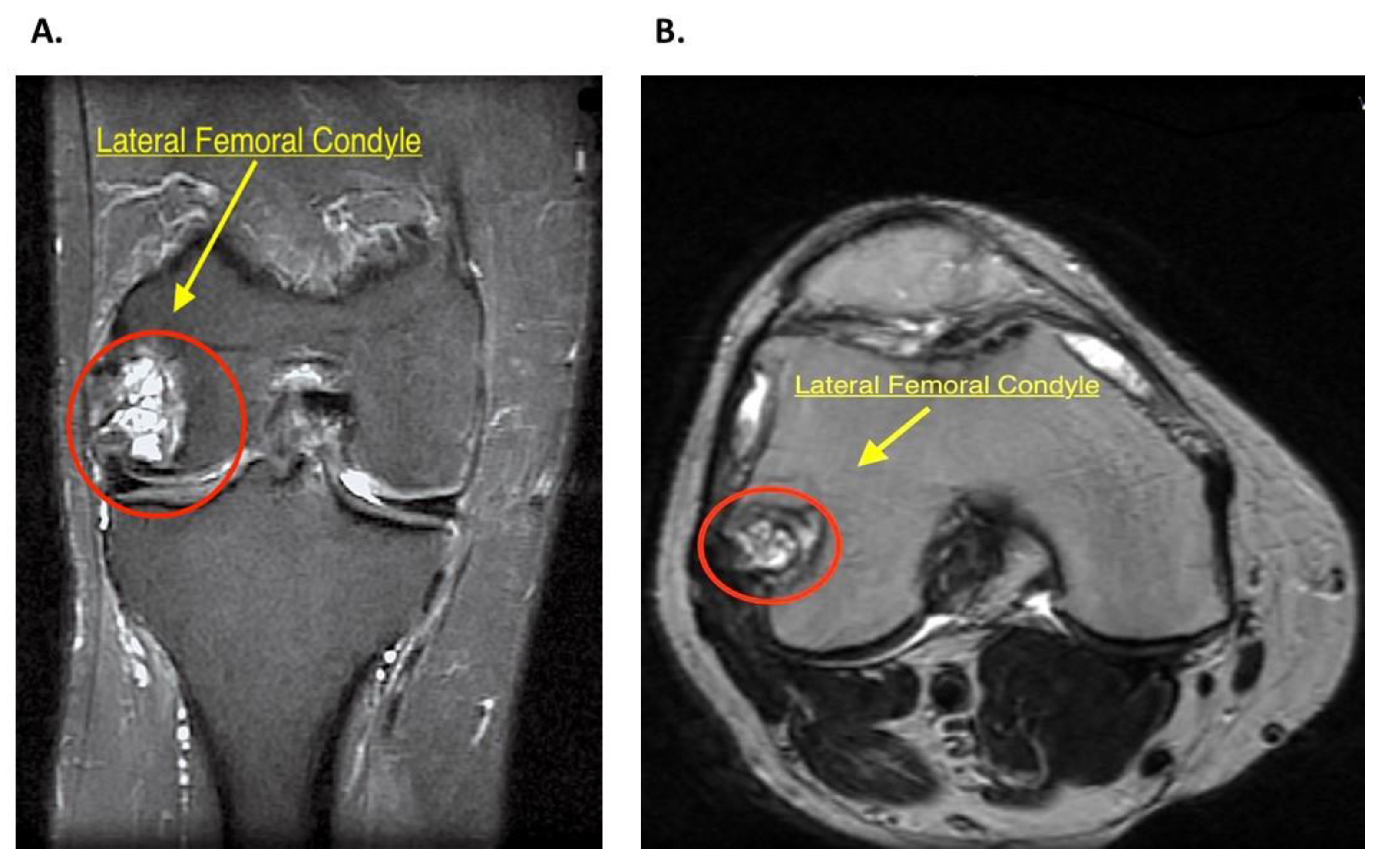The image consists of two grayscale scans against a black background, clearly depicting medical imaging, likely x-rays or CT scans, of a body part, potentially a knee. Each scan is labeled at the top with black text: the first image is marked 'A' and the second 'B'. In both images, there are prominent, thick red circles highlighting a white mass within the scans. These masses are identified by a yellow label that reads "lateral femoral condyle," with a yellow arrow pointing precisely to the circled area. The labels and arrows are consistent across both images, directing attention to the same anatomical structure but from slightly different angles, providing a comprehensive view of the lateral femoral condyles. The surrounding areas in each scan vary in shades of gray and black, typical of detailed medical imaging studies.